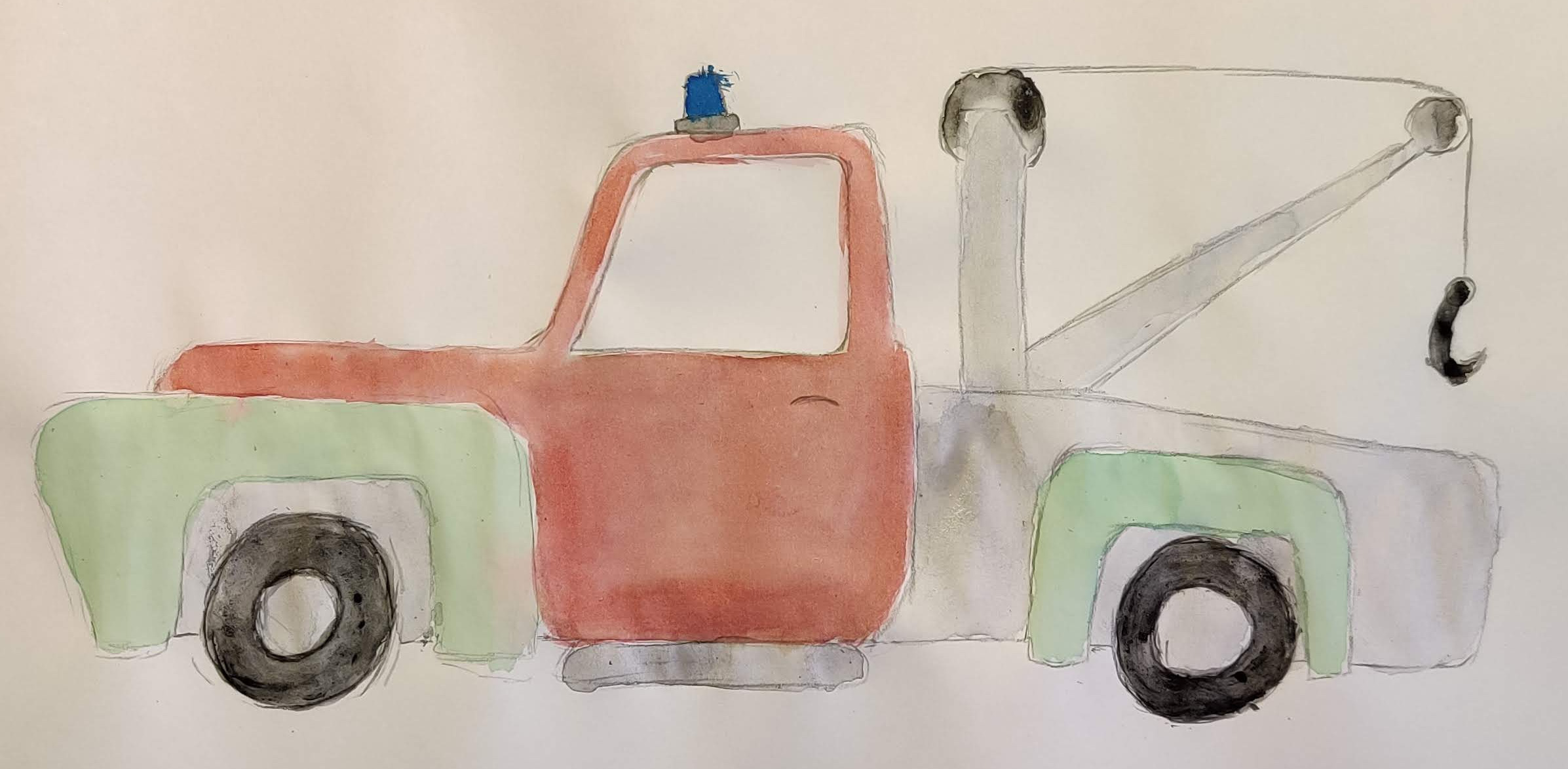This image features a detailed child's drawing of a tow truck on sketch paper. The truck is predominantly orange, and the artist used a pencil for the initial sketch before filling it in with watercolors. The truck's fenders are a sea-green color, while the tires are black. Atop the truck is a blue light, reminiscent of a police siren, indicating its emergency function. The truck includes intricate details such as the gray step-up ledge, a black hook on a gray winch at the back, and a well-defined handle for entry. The background and remaining parts of the truck are shaded in a very light white-gray, adding depth to the image. The level of detail and the use of mixed media, including pencil and watercolors, suggest a commendable effort, potentially by a child or teenager.